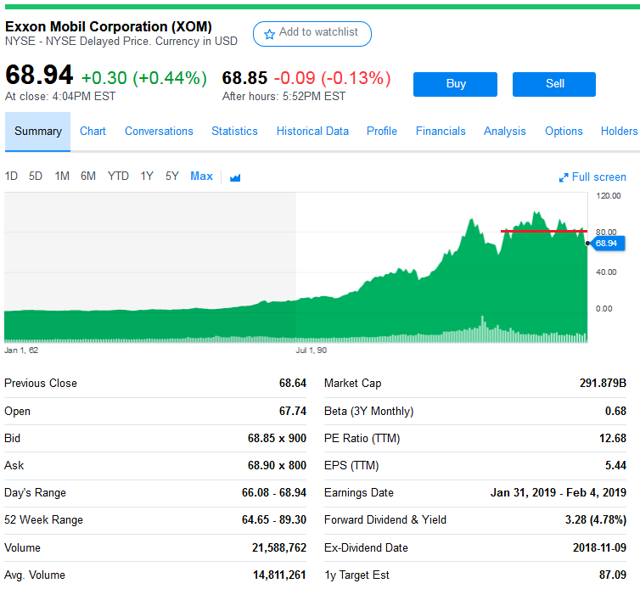A detailed and organized caption for the image described could be:

---
The image displays a comprehensive stock market chart for Exxon Mobil Corporation (ticker: XOM). In the center of the image, a green price chart illustrates the historical performance of Exxon's stock, highlighting a noticeable peak over time. To the left, various stock prices are listed, including the current price of $64.94, which represents a 0.44% increase, and the previous close at $68.64. Below these prices, additional trading details are provided: open price, bid, ask, day's range, 52-week range, volume, and average volume.

At the right side of the image, detailed market statistics are presented: 
- Market capitalization (291.879B)
- Beta
- Price-to-Earnings (P/E) ratio (12.68)
- Earnings Per Share (EPS) (5.4)
- Forward dividend yield (4.78%)

Additionally, the dividends are recorded at $67.74, with the upcoming earnings dates listed from January 31st to February 4th, 2019.

The overall design of the image is set against a white background for optimal clarity. The chart predominantly features green elements to indicate positive performance, with supporting text and data in white and black for enhanced readability.